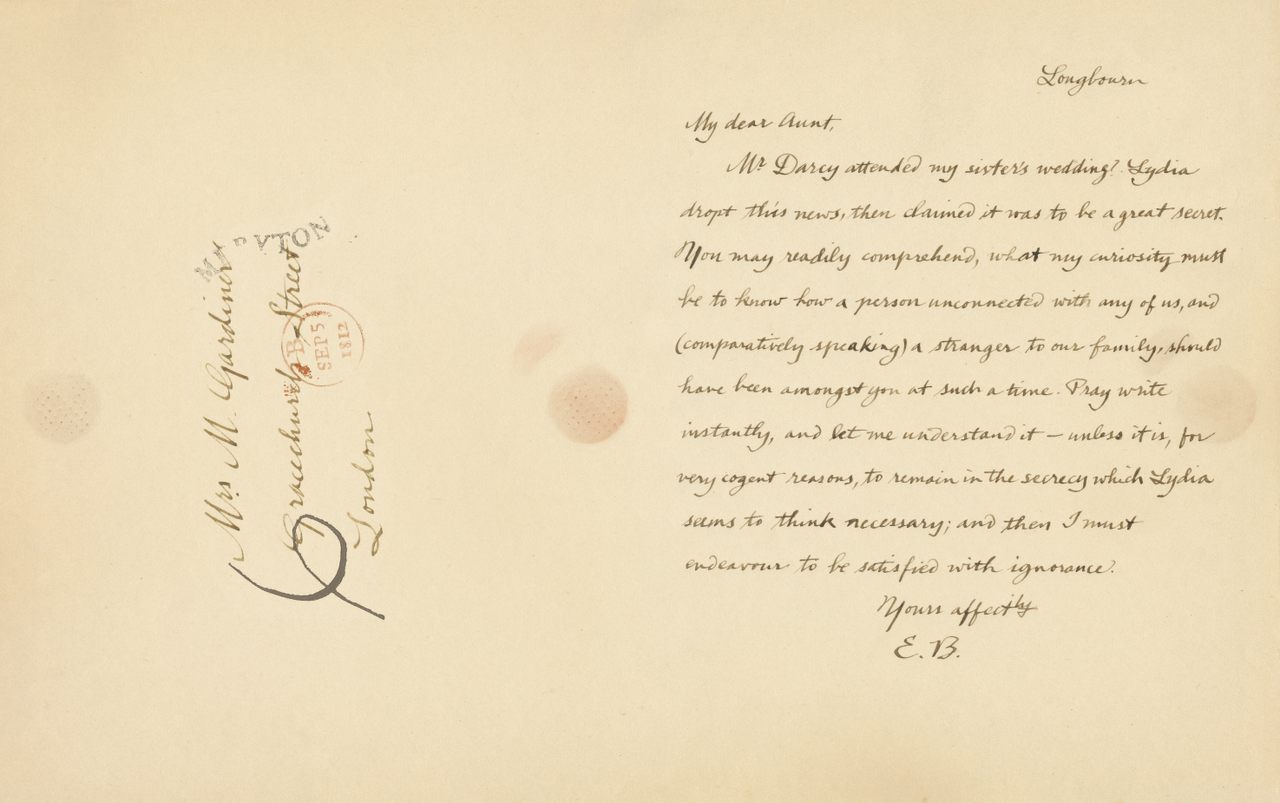The image features an aged, slightly pink-stained handwritten letter dated September 5th, 1812. The letter is penned in brown cursive script on yellowed parchment, suggestive of its considerable age. On the left-hand side, the recipient's address reads "Mrs. M. Gardiner, Grace Church Street, London." Notably, the name "Longbourn" appears at the top right corner. The body of the letter, addressed to "My dear Aunt," starts with the intriguing revelation that "Mr. Darcy attended my sister's wedding." The writer, E.B., expresses a fervent curiosity about how someone relatively unfamiliar and "unconnected with any of us" was present at the event, especially since Lydia had insisted the matter remain secret. The letter urgently requests an explanation, provided there are no compelling reasons for keeping it a secret. It concludes with "Yours affectionately, E.B." The overall wear and historical details of the letter enhance its authenticity and the sense of a long-passed era.